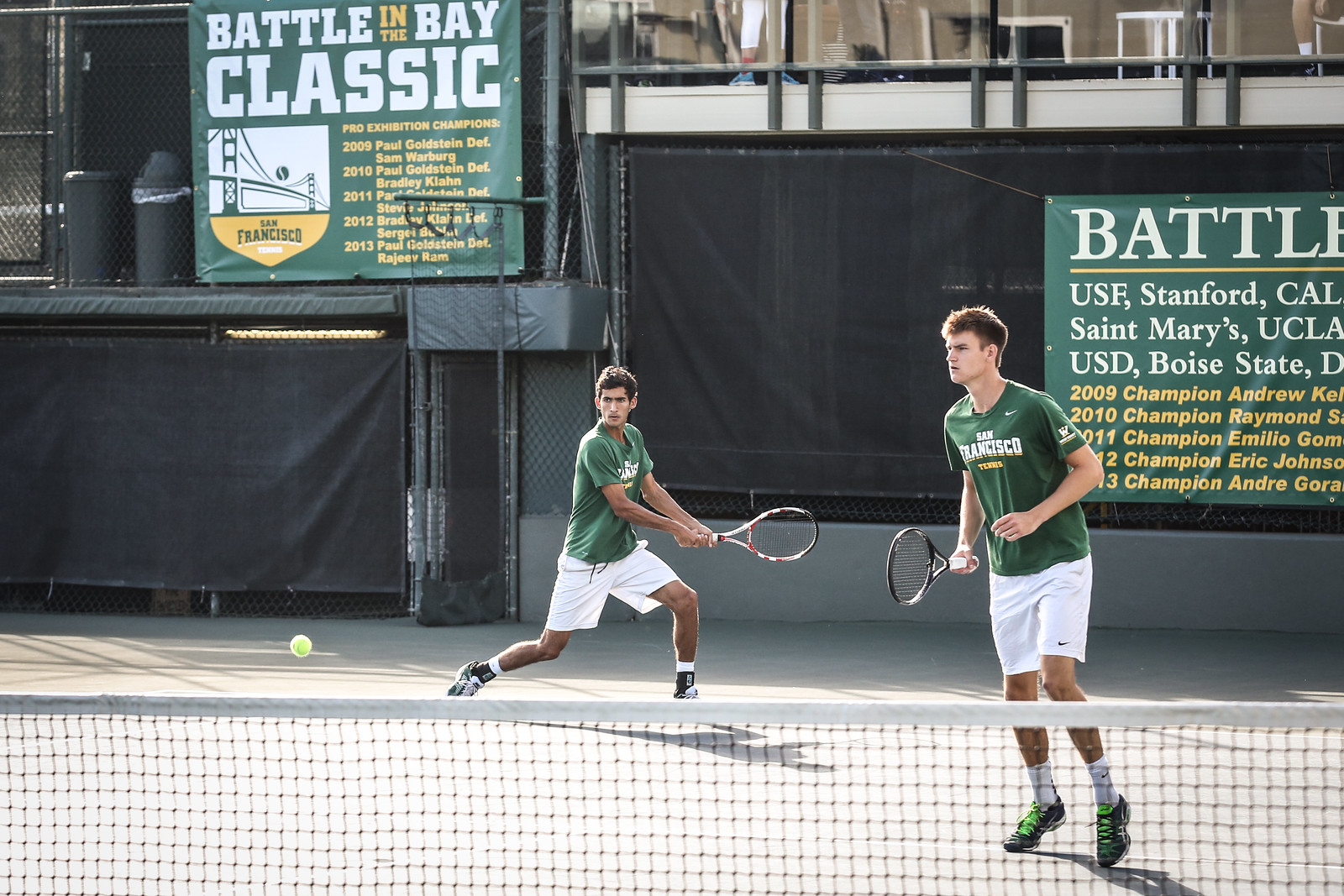In this dynamic outdoor daytime photograph, two tennis players in their teens or 20s are energetically engaged in a match. Both athletes are dressed similarly in green short-sleeved shirts and white shorts, complemented by black shoes, and they seem to be teammates positioned on the same side of the court. The player on the right, who appears to be of Caucasian descent with short brown hair, is in a ready stance, intently observing the action. On the left, his partner, a player with brown skin and dark brown hair, is in the midst of a powerful backswing, eyes locked on the oncoming tennis ball.

The court’s net, spanning the width of the lower section of the image, brings focus to the players' positions, with the player on the right closer to the viewer. Behind them, the back wall of the stadium is adorned with two large green banners. The left banner prominently displays the title "Battle in the Bay Classic" atop a shield featuring a bridge, presumably the Golden Gate Bridge, set against a white backdrop. Below the main title, additional details in yellow writing can be seen, though not entirely legible.

The right banner, partially cut off, reveals the word "Battle" and lists several prestigious universities and teams, including USF, Stanford, St. Mary's, UCLA, USD, and Boise State, indicative of a competitive collegiate event. Further down, golden inscriptions commemorate past champions with names like Andrew (2009), Raymond (2010), Emilio Gomez (2011), Eric Johnson, and Andre Cora.

Overall, this vivid image captures a moment of intense focus and athleticism, set against the backdrop of a notable tennis event celebrating collegiate talent and competitive spirit.